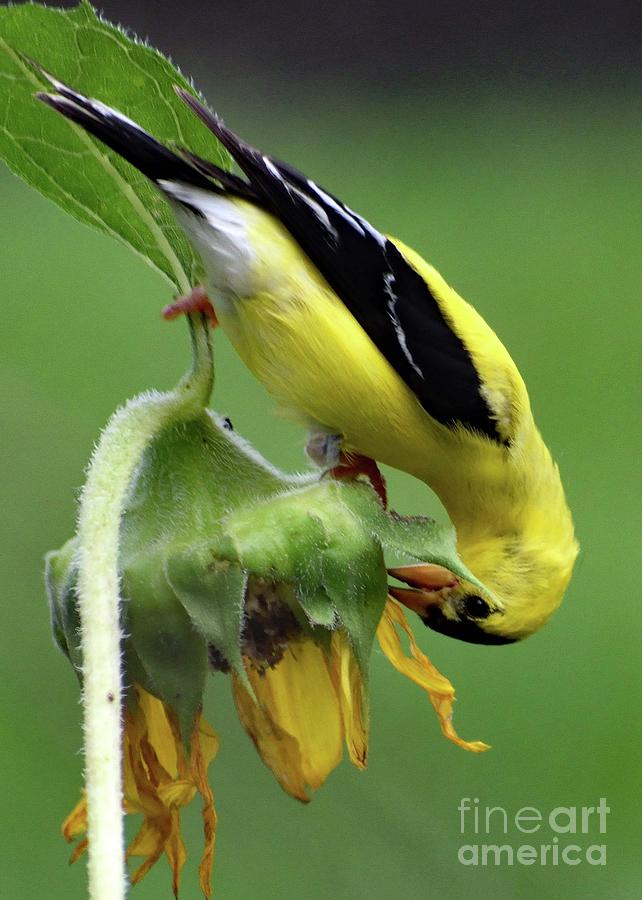In this captivating nature photograph, a slender goldfinch, exhibiting the characteristic yellow plumage with a distinctive black spot on its head, is seen in an intricate pose. Its forewings and tail feathers are adorned with touches of black and white, while its abdomen reveals a subtle white hue. The goldfinch is intricately perched atop a wilted yellow sunflower, which appears shriveled and dried, with a visible hairy stem. To extract seeds or perhaps an insect from the dying bloom, the bird has cleverly inverted itself, positioning its head upside down and leaning inward towards the flower. The background of the image is a blurred greenish tone with a hint of gray towards the top, creating a serene backdrop that enhances the finch's vibrant colors. In the bottom right corner, the image is signed in transparent white font with "Fine Art America," adding a touch of authenticity and artistic value.